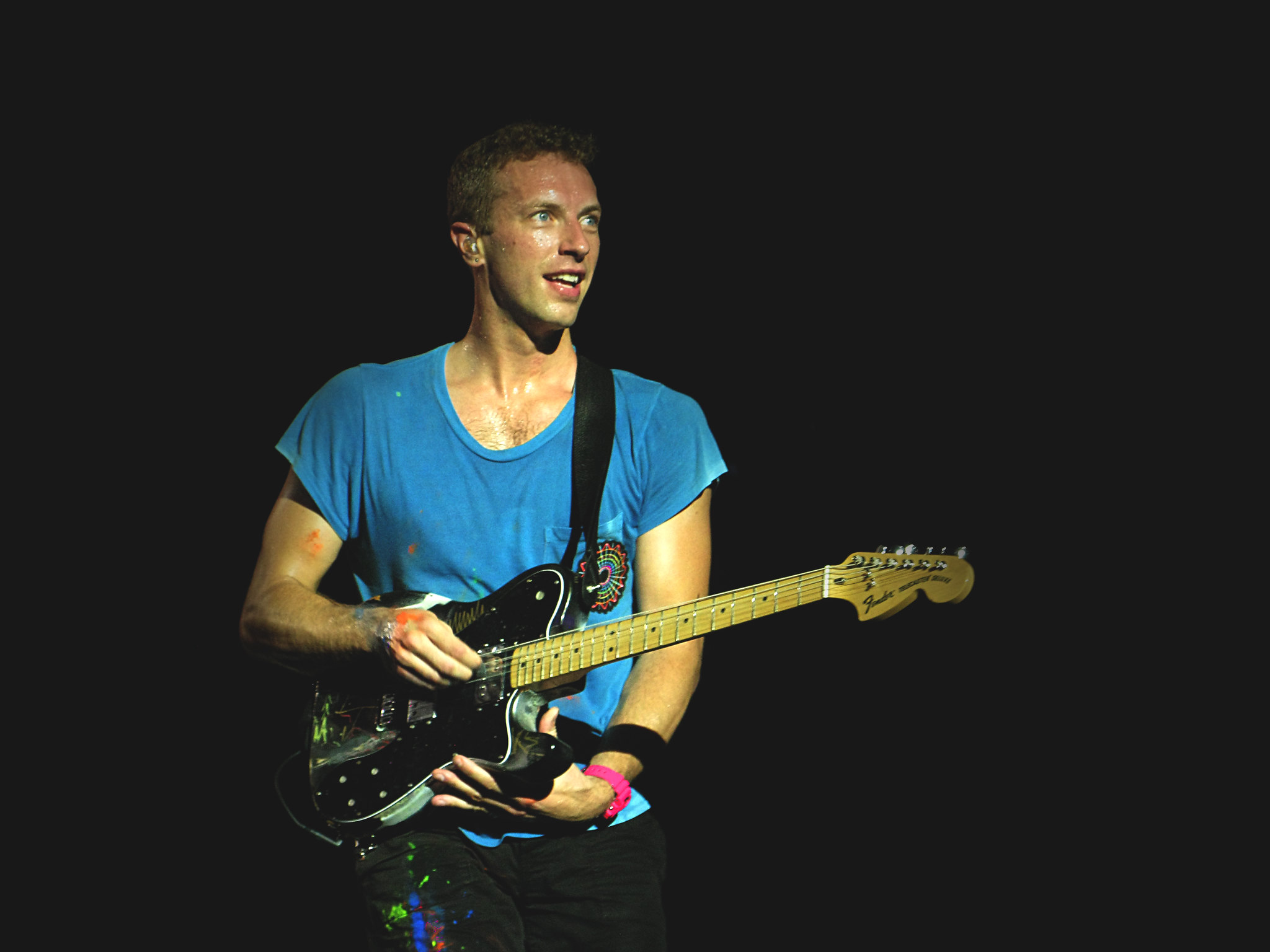The photograph features a male musician standing in a pitch-black background, illuminated by off-camera lighting from the right, highlighting the glistening sweat on his body, indicating the intensity of his performance. He is positioned with his shoulders squared to the camera, and his head turned to the right, where his open mouth suggests he might be mid-expression or mid-song. Cradled in his hands is a black electric guitar with a light brown neck, suspended by a strap over his shoulder. The musician is wearing a short sleeve blue T-shirt with a front pocket adorned with a rainbow-colored flower, and black pants splattered with random splashes of paint. His attire also includes a pink bracelet on one wrist and visible tattoos around his other hand. The photograph's stark contrast and lighting focus exclusively on him, leaving no other visible elements in the frame, thereby centralizing the viewer's attention on his intensely focused and energized presence.